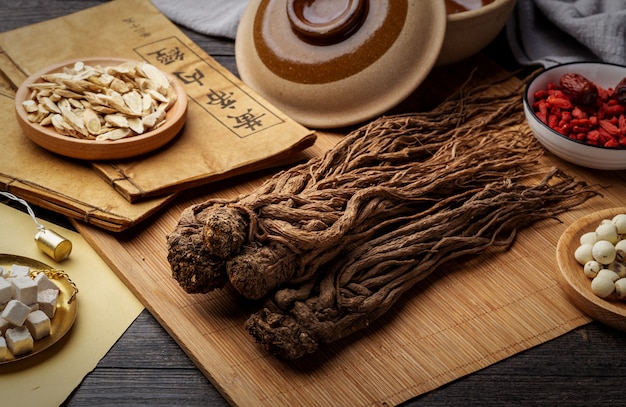The image displays an intricately arranged setting on a black wooden table, adorned with a bamboo-style placemat reminiscent of those used for sushi preparation. Central to the image is a curious, brown, stringy, and leafy object, possibly an herbaceous root or bulb, stacked in a trio. To its right rests a white porcelain bowl containing vibrant red, cut-up vegetables or seeds, with a date nestled among them. Adjacent to this, at the bottom right corner, is a wooden plate with small, white circular objects, possibly seeds or snacky foods.

Toward the upper left, a golden dish holds cube-shaped items that appear to be tofu or sugar cubes. Further back, there is a wooden plate with several brown objects, potentially seeds or nuts, which sits atop a book with Japanese or Chinese characters adorning its cover. An earthenware pot with its lid set slightly ajar is also visible, contributing to the photograph's intricate and eclectic arrangement.